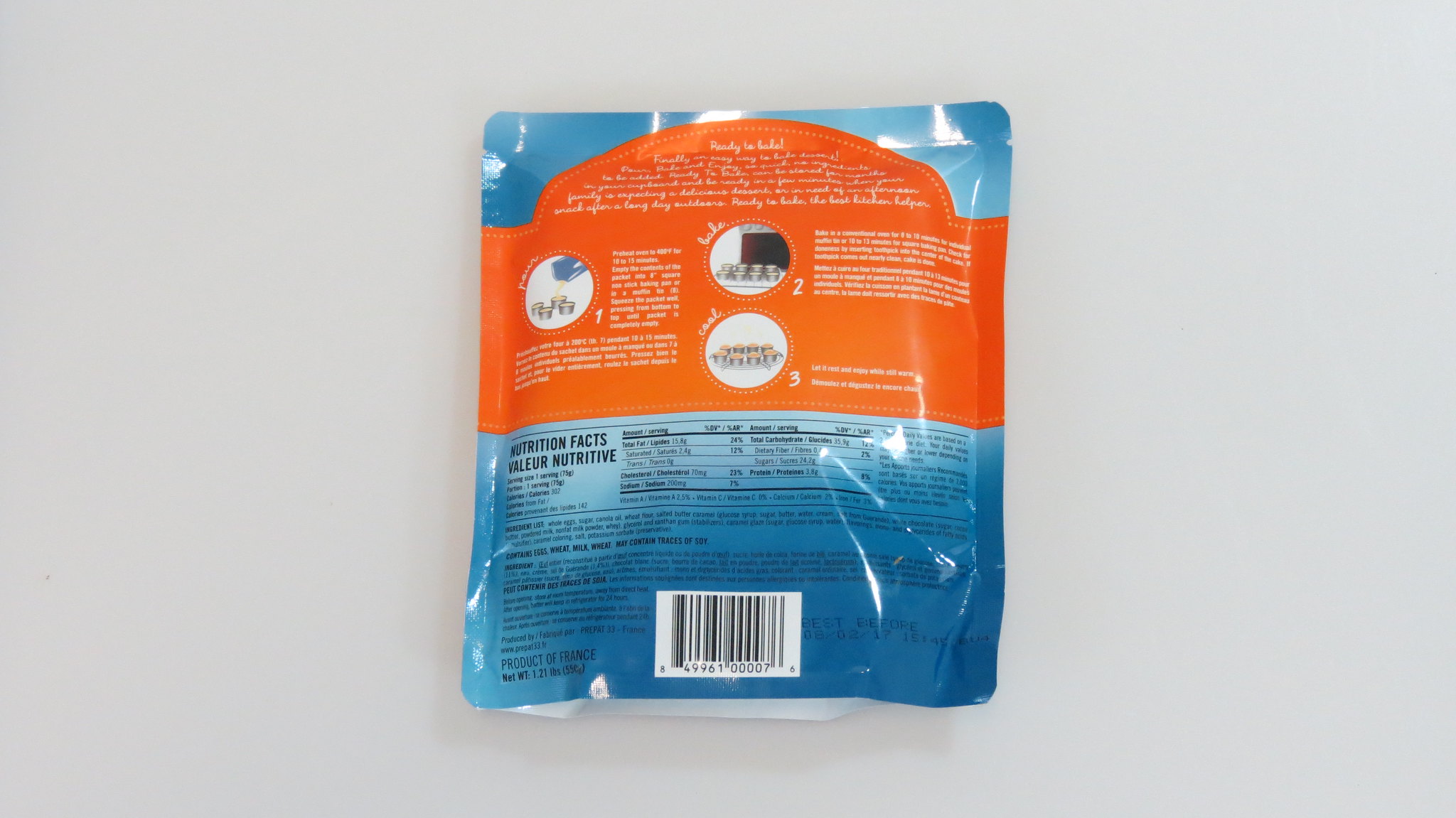This photograph depicts a glossy, blue plastic packet with a prominent orange section. The orange area features white text, while black text is printed on the blue portion of the packaging. At the bottom of the packet, there is a standard white and black barcode. Although the text is small and somewhat difficult to read on the orange section, the blue part near the bottom clearly displays "Nutrition Facts" and the French equivalent, "Valeur Nutritive." This indicates that the packet likely contains a nutritional supplement or food product. The packet is placed on a white background, such as a table, but without any additional objects or people to provide a sense of scale, it appears relatively small. The top of the package is perforated, designed for easy opening. The glossy surface of the packet reflects the light, highlighting its shiny texture.